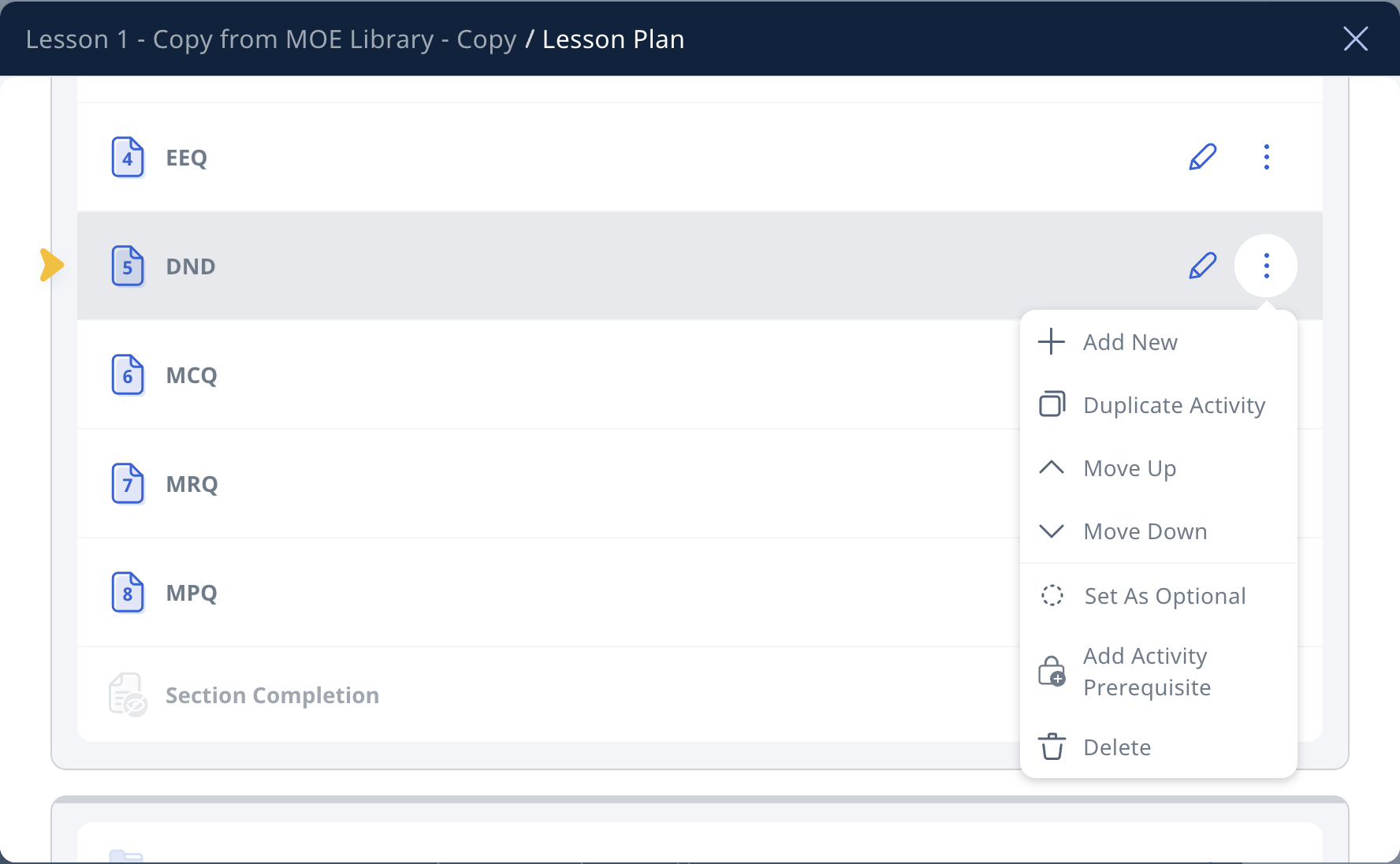Screenshot of an online lesson plan interface. At the top of the page, a black bar displays the text "Lesson 1 from MOE Library - Copy \ Lesson Plan." On the far right of this bar is an 'X' button, allowing users to close the window. Below the bar, there are five lesson plans listed in a vertical column, each represented by an icon of a paper with a folded corner.

1. **EEQ** - Marked with a paper icon and the number 4.
2. **D&D** (currently highlighted) - Marked with a paper icon and the number 5.
3. **MCQ** - Marked with a paper icon and the number 6.
4. **MRQ** - Marked with a paper icon and the number 7.
5. **MPQ** - Marked with a paper icon and the number 8.

To the right of the highlighted D&D lesson plan, there is a clicked three-dots menu displaying the following options:
- *Add New*
- *Duplicate Activity*
- *Move Up*
- *Move Down*
- *Set as Optional*
- *Add Activity Prerequisite*
- *Delete*

At the bottom of this section, "Section Completion" is displayed lightly, suggesting this area is related to tracking or setting the completion status of the section.